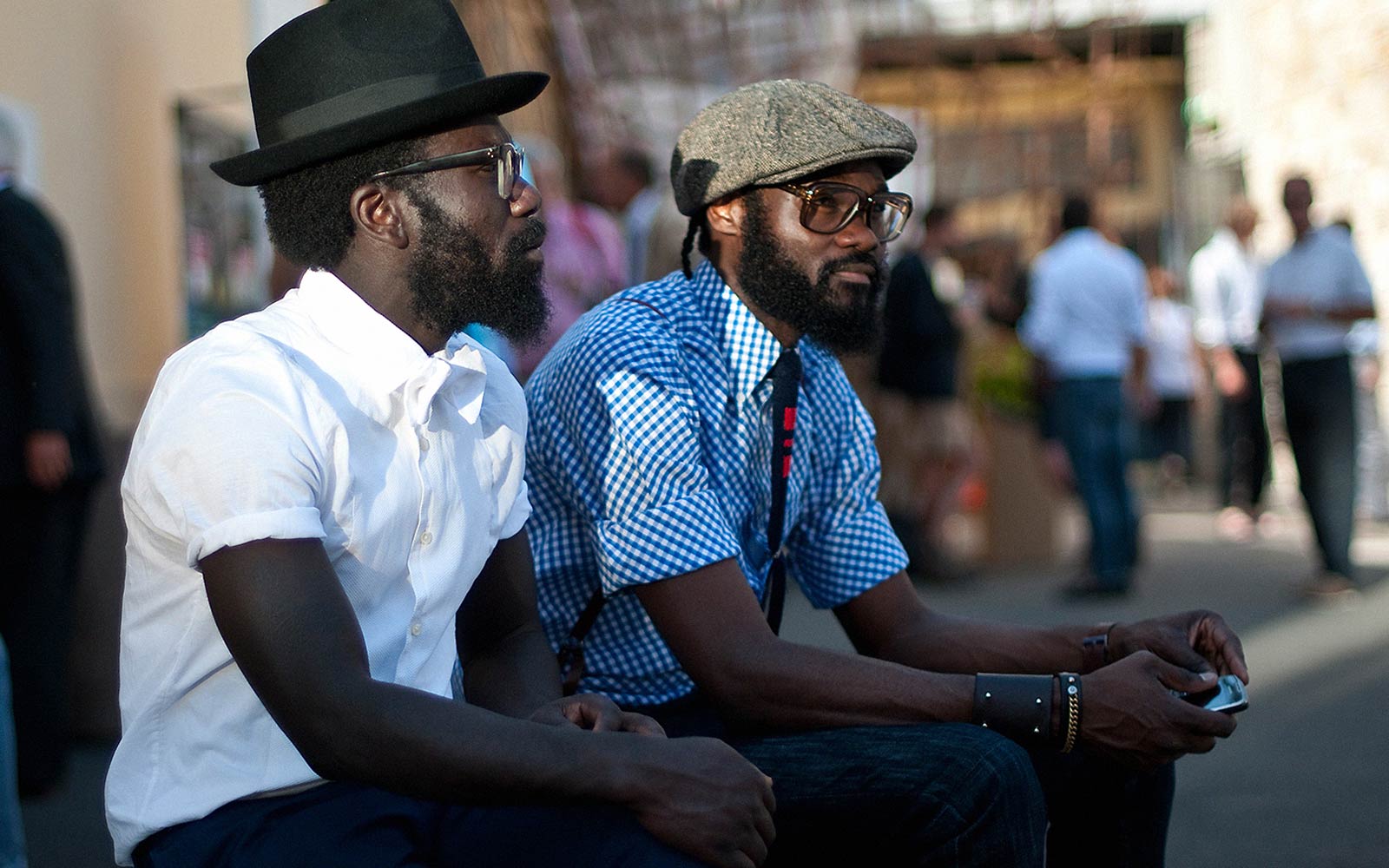This horizontally aligned photograph captures two African or African American men in their late 20s, exuding a hipster vibe. Both men, sporting dark brown skin, beards, and spectacles, are seated and facing mostly to the right, their arms relaxed in their laps. The man on the right, visible more from the front, wears a blue and white plaid short-sleeved button-up shirt with the sleeves rolled up, paired with a striking dark blue necktie adorned with red squares and a smaller red rectangle. He accessorizes with a thick leather wristband with four studs forming the corners of an imaginary square, a copper chain on a leather strap further up his wrist, and possibly another leather band on his other wrist. His light gray beret complements his black beard and mustache, and he's holding a cell phone in his right hand.

The man on the left, slightly looking up, dons a black fedora with a ribbon around the crown, a curly black hairdo, and a white button-up shirt buttoned all the way up, accented by a white bow tie. He's seated in blue pants, mirroring the relaxed posture of his companion with his elbow bent at roughly a 160-degree angle. 

The background features a blurred cityscape with low, ornate buildings reminiscent of the 1920s. A two-story building with yellow walls and square-shaped windows stands out on the right, while a pink cloudy-looking wall and several other structures add depth to the scene. A few blurred figures populate the backdrop, primarily concentrated on the left, where a man in dark pants and a light button-up shirt, with sleeves rolled up, is visible. Behind him, another man in similar attire appears with blonde hair, and a person in blue jeans stands facing away from the viewer.

Overall, this photograph, potentially taken in an urban area like New York within the last 15 years, showcases a dynamic, sunlit street scene with a focus on the two stylishly dressed men, surrounded by the blur of city life.